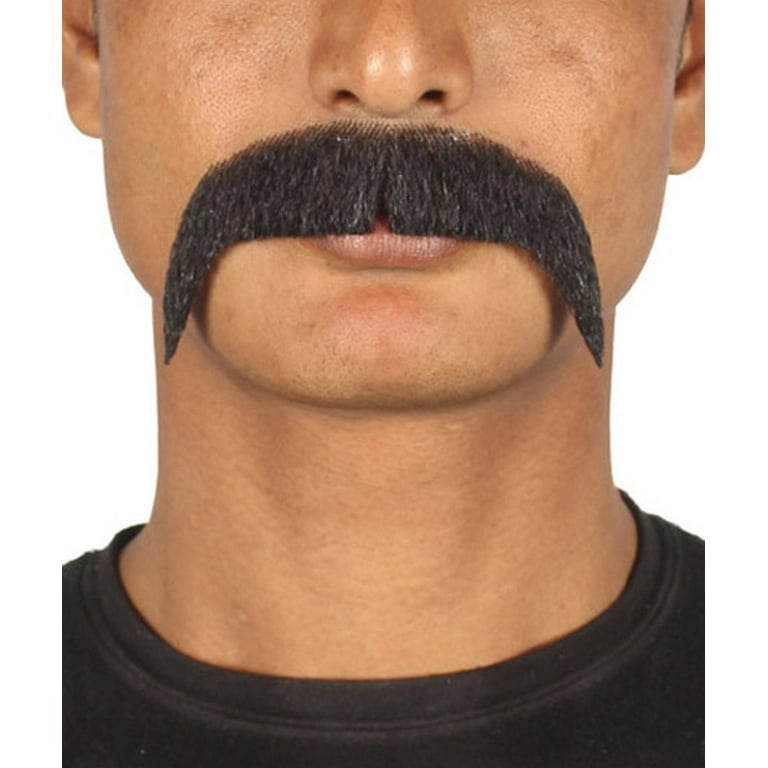This detailed photograph showcases a close-up view of the bottom half of a white male model's face, centered around his meticulously groomed large mustache, which extends across his upper lip and curves down the sides of his mouth. The background is stark white, likely edited to eliminate any distractions, thus emphasizing the focus on the model and the mustache itself. This type of presentation suggests a commercial or product photography setting, typical for online shop listings or catalogs. The image is tightly cropped, only showing the model from the upper half of his nose to just below his neckline, where he is wearing a dark brown or black crew neck t-shirt. The mustache appears strikingly well-groomed, possibly even a fake mustache made of coarse fabric or hair, giving the impression it could be a prop used in movie productions. The model’s skin is flawless and has a pinkish hue around the lips with a caramel undertone. The overall composition centers the mustache, slightly above the midpoint of the frame, with the neck and collar of the shirt filling the lower portion, and hints of the model’s ears appearing on both sides towards the upper part of the image.